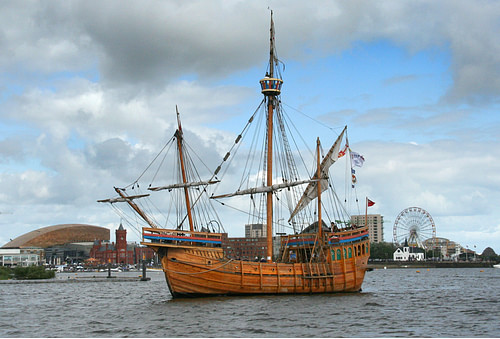The image captures a single galleon in the water near what appears to be a theme park or an area with similar attractions on the adjacent land. The land features a prominent giant ferris wheel on the right side near a white building with a pointed black roof, reminiscent of a schoolhouse or church. Behind the galleon, slightly to its right, a red flag is visible. The ship itself is made of a bright reddish-brown wood, with the majority of its sails closed and the masts appearing bare except for the lines and cables. On the left of the frame, a tall red building with a pointed roof, emitting a greyish hue from a distance, can be seen. The scene is complemented by birds flying close to the ship and a backdrop of a clear sky with some clouds.